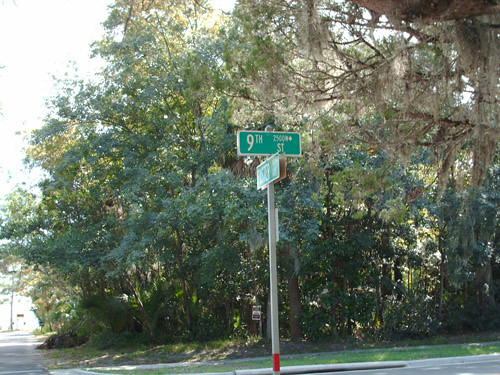This detailed color photograph captures an intersection with a prominent street sign at the side of the road. The signpost, gray with a red base, supports two green rectangular street signs with white text and borders. The top sign reads "9TH" (Ninth Street) along with an indiscernible number and a small diamond symbol to the right. The lower sign, oriented perpendicular to the top one, has illegible text. 

In the background, a lush scene unfolds with a green lawn, gray asphalt or sidewalk extending to the left bottom corner, and dark green bushes sprouting from the grass. Various trees, both tall and short, fill the scene. Most have green leaves, but one particularly tall tree to the photo's right stands out with white leaves and light brown, tan-colored moss hanging from it, adding a unique texture. The interplay of greenery and the street signs anchors the scene in a tranquil, yet well-defined urban landscape.